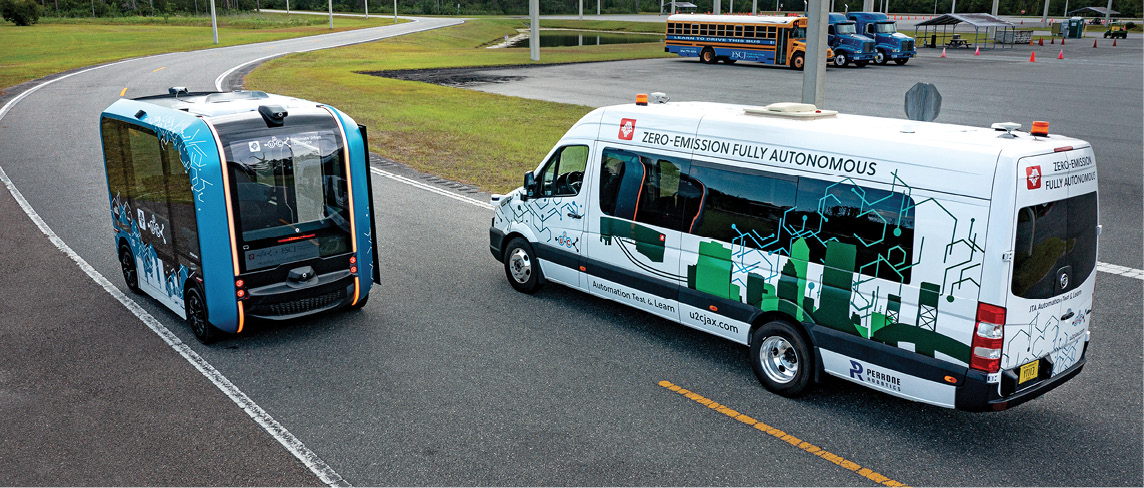The image depicts a scene on a curving two-way street populated with two distinctive autonomous buses. The vehicle closest to the camera is a white van adorned with green lettering and advanced blue and green graphics, including illustrations of chemical symbols and a cityscape. This white van, marked with messages like "zero emission," "fully autonomous," and "automation test and learn," references the website use2seejax.com. The other vehicle, further down the road and traveling in the opposite direction, is a smaller, almost rectangular, teal-blue bus with orange highlights and red lights. Both buses appear to be self-driving, futuristic transport solutions with zero emissions. In the background, a row of standard school buses can be seen, including a mix of blue and orange buses, parked near an awning with a bench. Orange cones are placed in the parking lot, possibly as safety measures around the autonomous vehicles. The detailed markings and unique shapes of these buses make them stand out against the typical street setting.